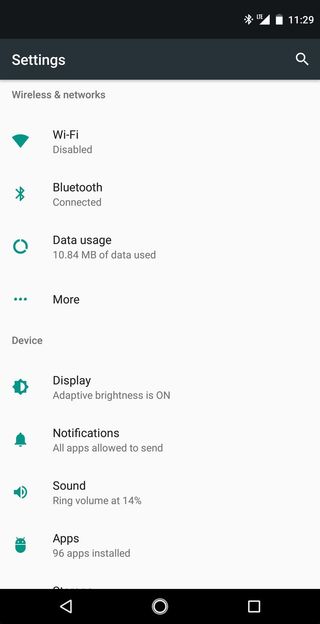This is a detailed screenshot captured from a tablet or smartphone. The screen is surrounded by a dark black bezel at the top. On the right-hand side of this bezel, there is a white Bluetooth symbol, followed by a cell phone signal indicator displaying "LTE," which is not full. Next to it is a nearly full battery icon. The time displayed is 11:29. 

On the left-hand side, there is a dark gray bezel with the word "Settings" in white, A magnifying glass icon is also shown in white on the right-hand side of the gray bezel.

The main content of the screen is organized in a white area with various icons and text. The first section, titled "Wireless and Networks" in gray, has a teal-colored Wi-Fi symbol next to bold black text reading "Wi-Fi." Underneath, in gray text, it states "Disabled." Following this is a teal Bluetooth icon, next to which is the word "Bluetooth" in bold black text, followed by "Connected" in gray.

Further down, there is a teal-colored circle symbol indicating "Data Usage" with bold black text to the right. Underneath, it reads "1084 MB of data used" in gray. A section labeled "More" is marked by three teal ellipses and the text "Device" in gray underneath.

Next, there is an image of a sun, split into teal and white halves, with the sun itself in teal color. The bold black text "Display" is found beside it, and below this, in gray, it reads "Adaptive brightness is on." 

Following sections include various settings options:
- A teal bell icon with the text "Notifications" in bold black, and below it, "All apps allowed to send" in gray.
- A teal speaker icon labeled "Sound," with "Ring volume at 14%" in gray.
- An Android character icon denoting "Apps," with "96 apps installed" stated underneath in gray.

There is another section visible but partially cut off. 

On parts of the screen and interface, the dark black bezel of the phone reappears, and at the bottom, navigation icons are displayed: a white overturned arrow pointing left, a white circle, and a white square.